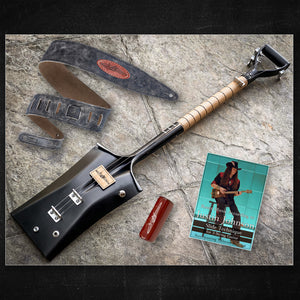This image captures a top-down view of several items arranged on a mostly tan and gray tile floor with some streaks. On the upper left side lies a twisted belt-like object; it is black on the outside and brown on the inside, with an orange oval on top of it. Adjacent to the belt on the right is a shovel with a black head and a wooden brown handle. Further to the right of the shovel is a small red object. To the far right is a rectangular, dark teal music program featuring a man playing a guitar. The man on the cover is dressed in a black hat, black and red shirt, dark blue jeans, and brown boots. All items are arranged on the tiled floor, creating a visually intriguing composition of everyday objects and music memorabilia.